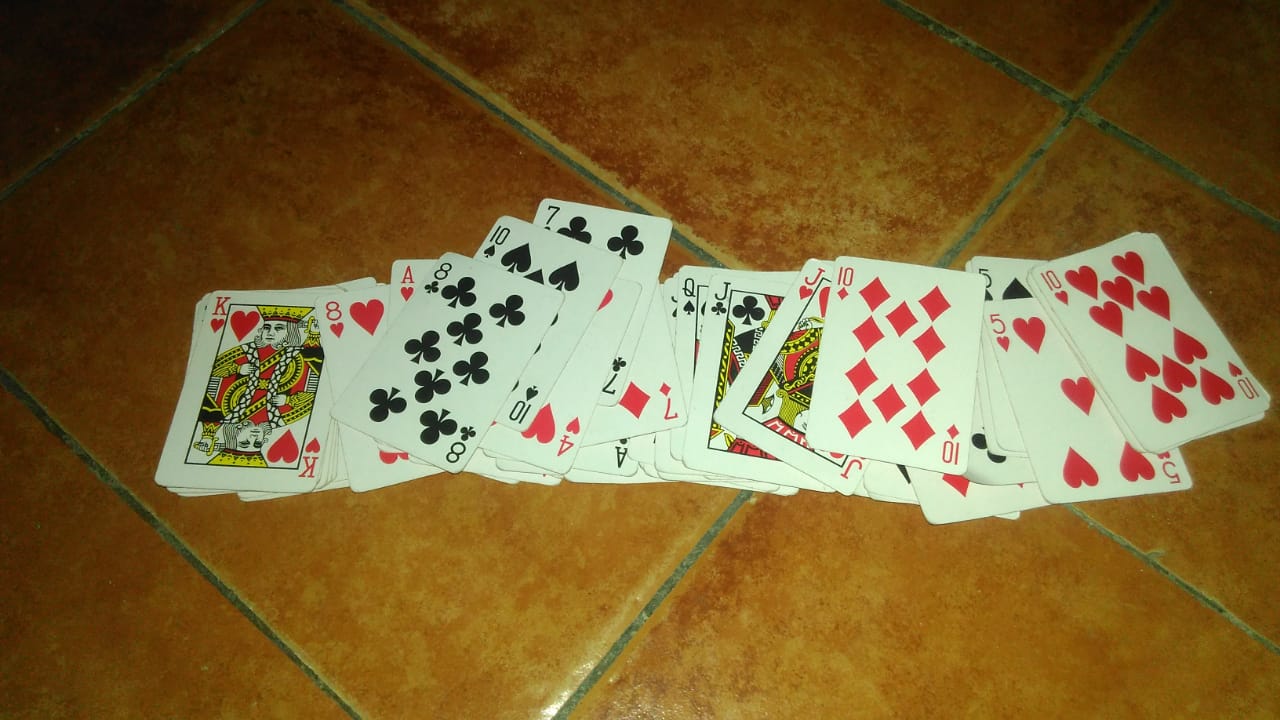The photograph features a scattered yet somewhat orderly pile of playing cards laid out on a floor composed of large, reddish-yellow tiles resembling bricks. These rectangular tiles are roughly uniform in size, separated by grayish grout lines. The visible section of the flooring comprises approximately 8 to 10 tiles, though the entire tile setting is cut off at the edges of the frame. The image itself is somewhat shaded and dark, exhibiting less-than-optimal quality with noticeable black spots near the top, likely due to shadows or insufficient lighting.

The cards are face-up and form two main stacks. One stack, towards the left side, sees the King of Hearts at the base, with an Eight of Hearts, an Ace of Hearts, an Eight of Clubs, a Ten of Spades, a Four of Hearts, a Seven of Clubs, a Seven of Diamonds, and an Ace of Clubs layered somewhat haphazardly over each other. The other stack, positioned more centrally, starts with a Queen of Spades, topped by a Jack of Spades, a Jack of Hearts, a Ten of Diamonds, an obscured card that is a Spade, a Five of Hearts, a Five of Spades, and finally a Ten of Hearts. Despite the apparent disarray, the cards in both stacks are neatly arranged one on top of another, each stack forming a somewhat orderly pile.